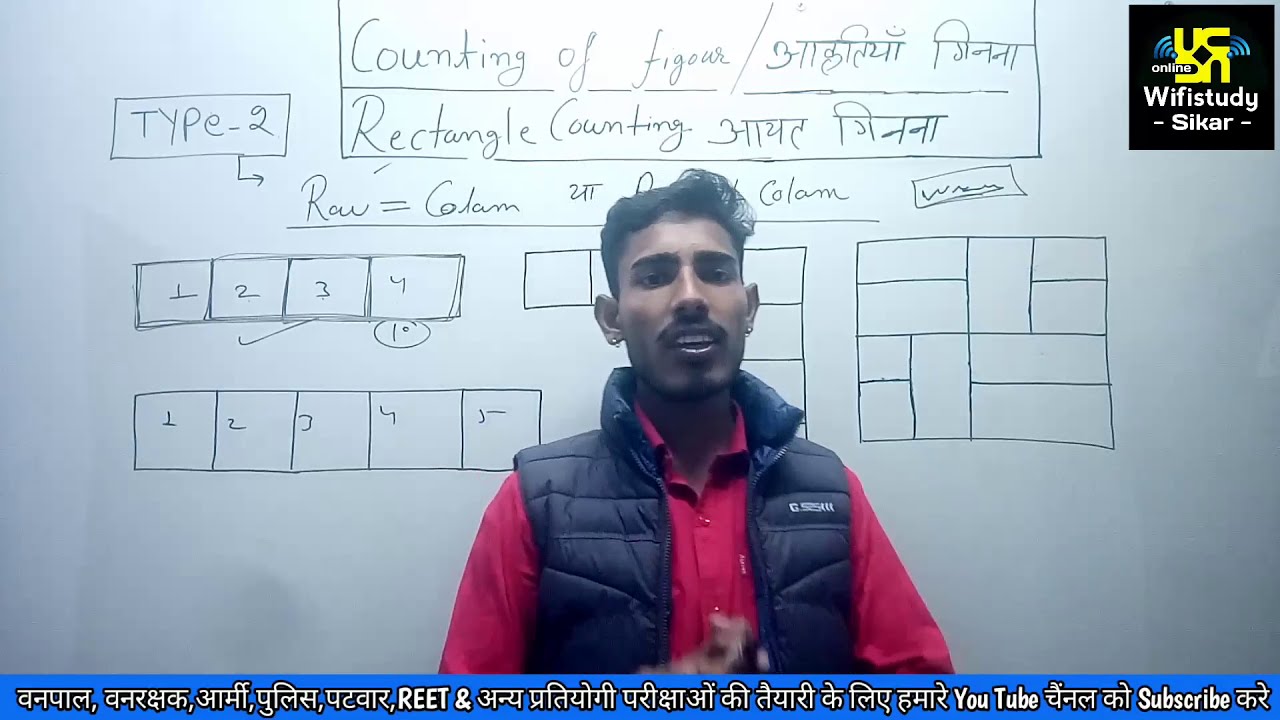The image depicts a young Indian instructor, likely in his mid to late 20s, teaching or tutoring about counting on a whiteboard. The instructor, wearing a red button-down shirt and a sleeveless black puffer jacket, has black hair, black facial hair, and earrings. He is speaking, with his mouth open and the top row of his teeth visible, and his camera has a faint light flare at the top.

Behind him, the whiteboard is filled with detailed annotations and diagrams. At the top, it reads "counting of figure, rectangle counting" along with some Hindi text. Various shapes and boxes are drawn on the whiteboard, resembling a maze, with additional text such as "type-2," "row = column," and "W with a squiggle." There are rows of squares arranged in patterns and an amalgamation of smaller squares forming a larger one. An arrow pointing to the right is also depicted on the left side of the board.

In the top right corner of the image, there's a yellow square symbol composed of rotated and mirrored letters "U" forming a pattern, with a diamond cut-out in the center. Below this symbol, it says "Wi-Fi study, SIKAR" and "online" within the opening of a reversed "C." At the bottom of the image, there is a blue caption bar with text in an Indian language, along with legible words like "YouTube" and "subscribe."